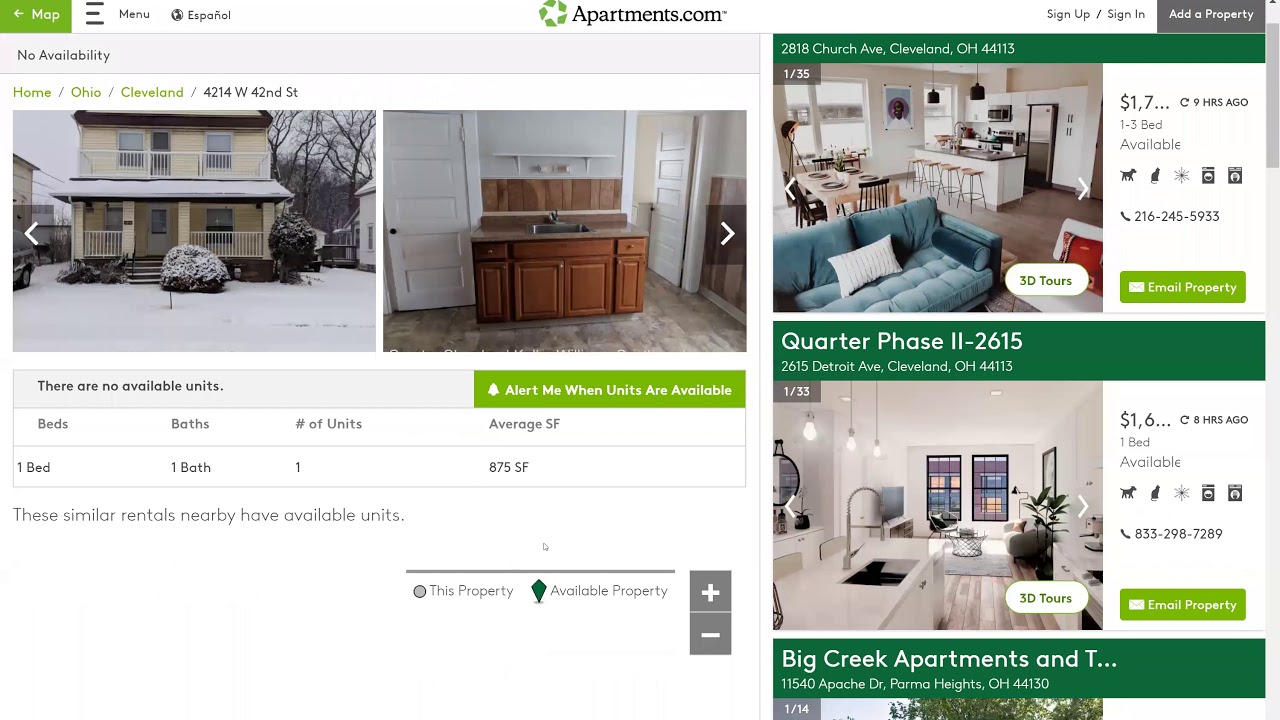The image is a screenshot from Apartments.com. At the top center of the image, the Apartments.com logo can be seen, featuring the text "Apartments.com" in gray alongside a small green circle composed of leaf-like shapes. The site clearly displays listings from Cleveland, Ohio, as indicated in the upper left-hand corner. The primary listing focuses on an address: 4214 West 42nd Street.

This specific listing includes several photos. The first is an exterior shot of a two-story, light yellow house with a frame structure, set against a snow-covered front lawn, establishing a sense of the surrounding environment. The second photo captures part of the kitchen, highlighting the sink accompanied by brown wooden cabinets underneath. 

On the right side of the screen, two additional images are presented. The first showcases a living room featuring a cozy blue sofa and a kitchen bar equipped with several bar stools. The photo beneath this one illustrates an open floor plan where the kitchen is seen in the foreground, and the living room is easily observable in the background, providing a glimpse into the spacious and connected layout of the interiors.